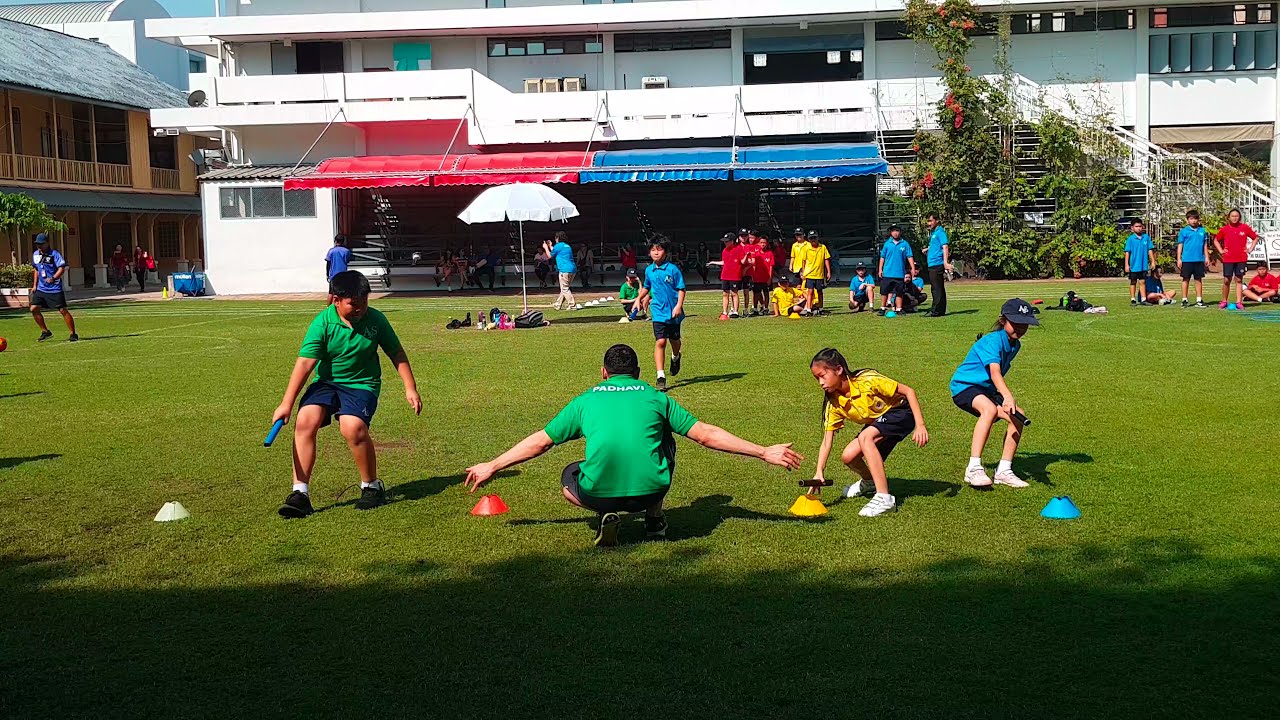In the image, there is a vibrant scene of South Asian children participating in a team game, possibly a baton race, on a green grass field. Three groups of students are distinguishable by their polo shirts—red, yellow, and blue—forming somewhat organized lines. In the foreground, an adult in a green polo shirt is squatting with his back to the camera, guiding three children who are reaching for colored cones or barriers on the ground. The child on the left is wearing a green shirt and blue shorts, the middle child wears a yellow shirt and blue shorts, and the child on the right has a blue shirt and dark blue shorts.

Behind the field, a large white building with white steps and two balconies stands prominently, adorned with a red and blue awning. To the left of the field, a brown building featuring a balcony can be seen. A single white umbrella is positioned in the distance near the white building. Various colored cones (white, red, and yellow) are scattered across the field, marking the game boundaries. A girl in a yellow polo shirt clutches a baton while reaching for the yellow cone, and another girl in a blue polo shirt also holds a baton, poised for action. Farther back, bleachers line the edge of the grass, dotted with more children in the background shadows.